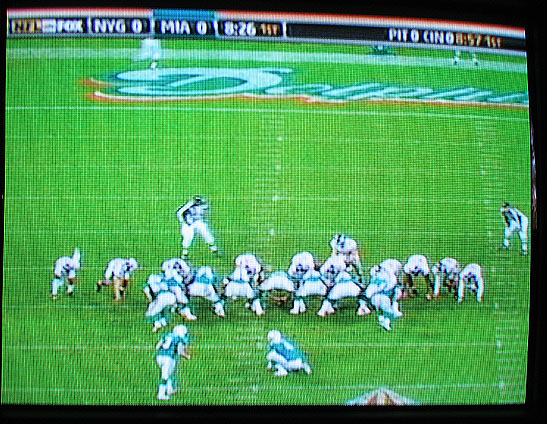This photograph captures a television screen displaying a live football match. The screen is surrounded by a sleek, reflective black border. On the field, two teams are playing; one team is dressed in green and white uniforms, while the other dons white and dark-colored attire. Two players are seen kneeling, possibly recovering or preparing for the next play. A referee is positioned in one corner of the screen. The lush green grass of the field is clearly visible, along with crisp white markings indicating various zones and boundaries. End zone markings in white and green are also discernible. Displayed at the top of the screen is the "NFL on Fox" logo, along with a current tie score of 0-0. The image quality is decent, making the details of the match easy to see.